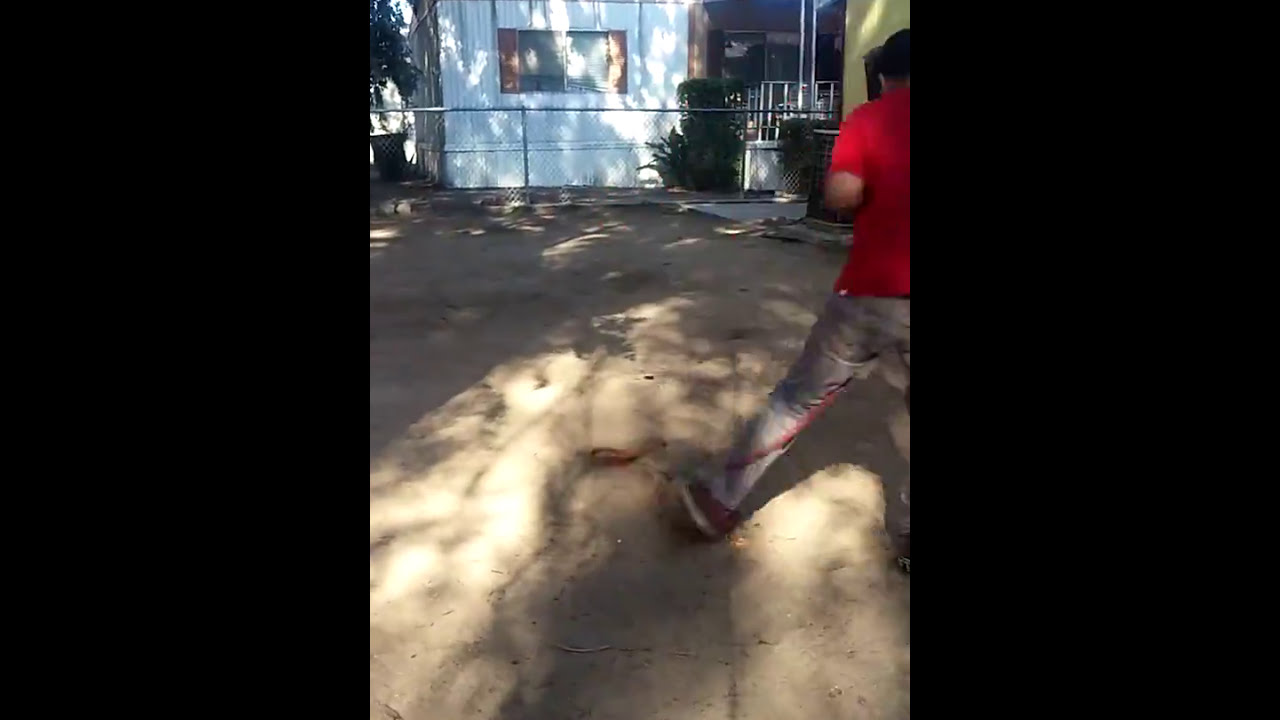The image, vertically divided into three sections with the left and right portions entirely black, features a central outdoor scene. Dominating the foreground, a man stands with his legs slightly apart, wearing worn, holey gray jeans and sneakers with white soles. His back, clad in a red short-sleeved t-shirt, is turned towards us, and he appears to be mid-step. He has dark hair. The man stands on a large concrete platform, surrounded by a chain-link fence that curves leftward towards the top of the picture, enclosing the area. Beyond the fence, a blue building with a large picture window, a porch, and a yellowish-green wall can be seen. The scene is dotted with plants, trees, and bushes, contributing to the rundown, slightly neglected atmosphere of the setting.